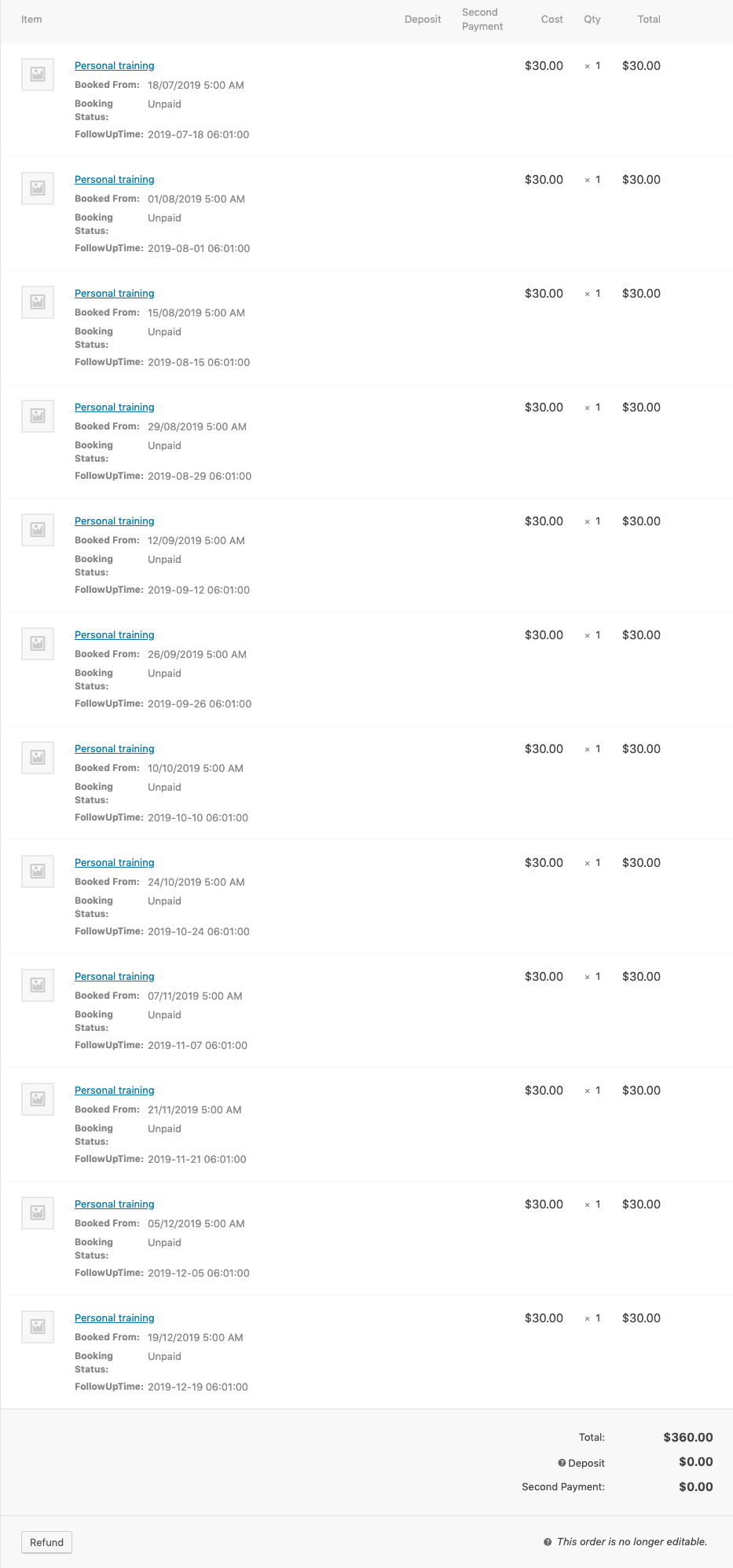The image depicts a document related to personal training sessions. The main section lists entries for individual training sessions, each with details such as the date of the session, payment status, and cost. Specifically, each session costs $30, with a running total of $30 per session. There are twelve sessions listed in total, significantly contributing to the overall amount.

The text is primarily in black on a white background, with the phrase "Personal Training" highlighted in blue at the top. Toward the bottom, the document shows a grand total of $360, with no deposit indicated, and possibly some mention of zero-dollar transactions, though the text is mostly unreadable.

In the bottom left-hand corner, there is a button labeled "Refund." Additional text is present in the bottom right corner, indicating the order status, but it is extremely small and difficult to decipher clearly.